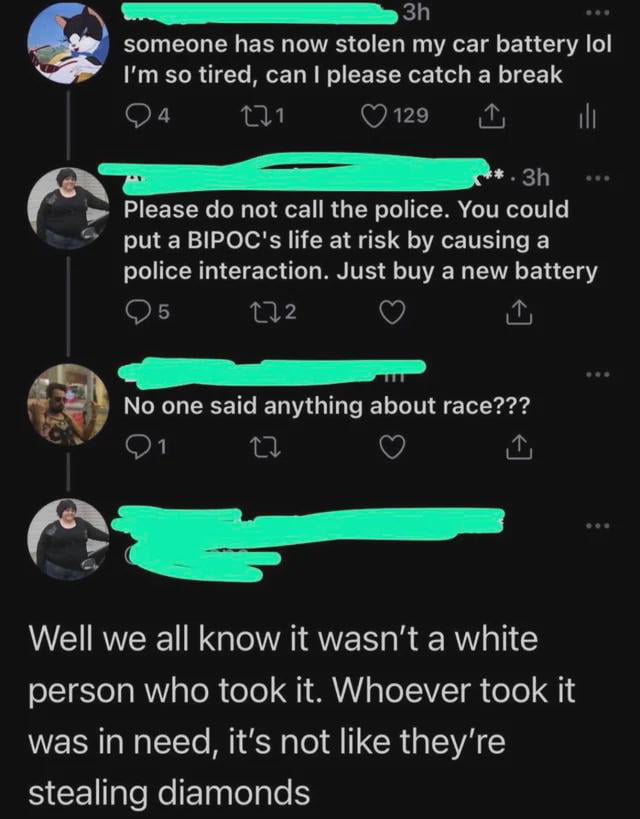This is a screenshot of a chat conversation among three users, with their IDs or handles obscured in green. The first message is from a user whose avatar depicts a cartoon cat. They express frustration, writing, "Someone has now stolen my car battery lol I'm so tired can I please catch a break." The second message comes from a user with an avatar of a heavyset white woman with short dark hair. They advise, "Please do not call the police you could put a BIPOC's life at risk by causing a police interaction just buy a new battery." The third message is from a user whose avatar shows a young man wearing sunglasses, possibly seated in an office. They respond incredulously, "No one said anything about race???" The second user replies, "Well, we all know it wasn't a white person who took it, whoever took it was in need, it's not like they're stealing diamonds."

The entire conversation is visually marked by the avatars associated with each user and the unique context provided by their differing perspectives.